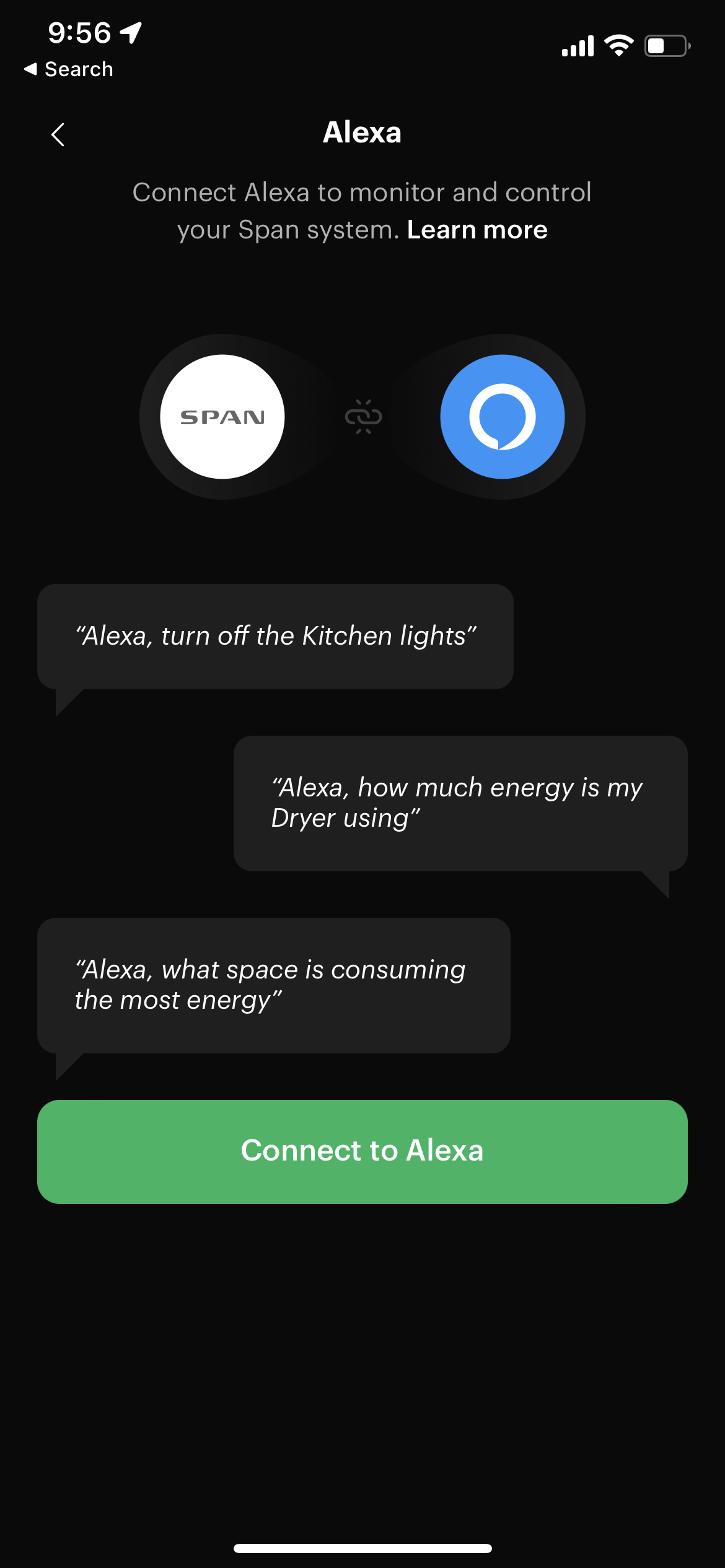Screenshot of a mobile device, possibly an iPhone or Android, in dark mode. The background is completely black. The time displayed at the top is 9:56, although it's not clear if it's a.m. or p.m. The device shows active location services, 4-bar cellular signal strength, 3-bar Wi-Fi strength, and a battery level at approximately 50 percent.

The top banner indicates an active conversation with Alexa, Amazon's AI assistant. It highlights the integration with the SPAN system for home energy management. The banner reads: "Connect Alexa to monitor and control your SPAN system." Below, in bold, it says "Learn more."

The chat interface demonstrates Alexa's capabilities:
- "Alexa, turn off kitchen lights."
- "Alexa, how much energy is my dryer using?"
- "Alexa, what space is consuming the most energy?"

This indicates Alexa's ability to manage and report on home energy efficiency, control electrical appliances, and provide detailed energy consumption information.